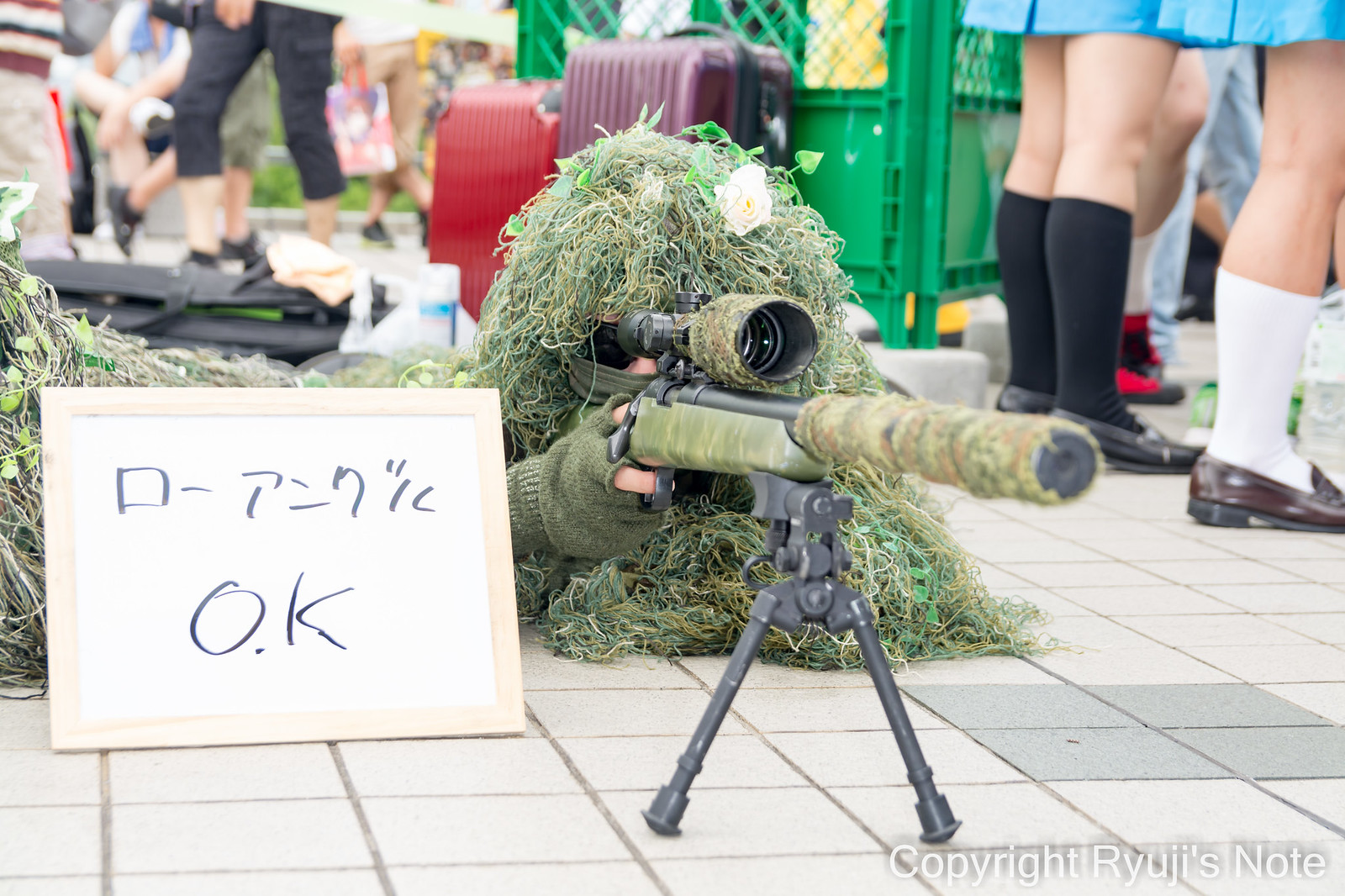In a striking juxtaposition, the image portrays a person in a meticulously crafted military ghillie suit, designed for extreme camouflage with an array of foliage and even a solitary flower, lying on the ground. They are adorned with green wool fingerless gloves, a matching green scarf, and sunglasses, accentuating their covert appearance. The individual is looking intently through the scope of a black-barreled rifle, which is camouflaged with vegetation and supported by a black bipod. 

In front of them, a white dry erase board with a light brown border displays handwritten Asian characters and the acronym "OK." The setting features a ground paved with small cement tiles, with noticeable grouting in between. 

To the right, several pairs of legs are visible, clad in knee-high socks—some white, some black—and blue skirts, indicating the presence of schoolgirls. Further in the background, additional figures are faintly visible, some wearing black trousers. The incongruity of the camouflaged individual in the paved environment, amidst casually dressed people, adds an intriguing layer of contrast to the scene.